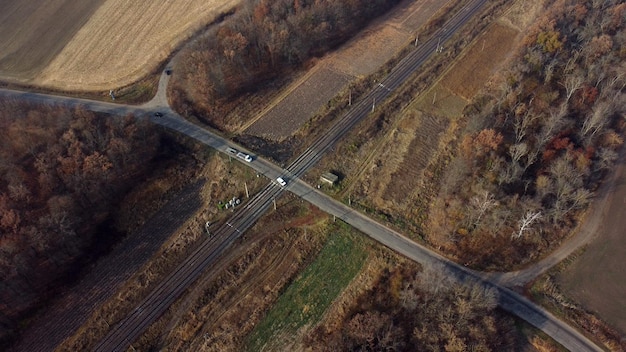This aerial daylight color photograph captures a rural intersection with a road and a railroad crossing. The main road enters the frame from the upper left, extending diagonally to the bottom right, intersecting with a double railroad track that comes in from the bottom left and stretches towards the upper right. A white car is visible crossing the railroad tracks, accompanied by two flatbed trucks behind it. The road also has curves branching off to the top and bottom of the image. Central to the image, at the crossing point, there's a small structure with a brown roof and a sliver of its white front visible.

Surrounding this intersection are various landscapes: wooded areas with trees showing autumnal hues of brown and orange or bare branches, fields that appear dry, and patches of flat brown dirt. Towards the bottom and middle right, there's a mix of green and brown flat areas, while the upper left features more expansive fields and brown trees. Additionally, power lines are seen following the railroad track's path, accentuating the rural setting.